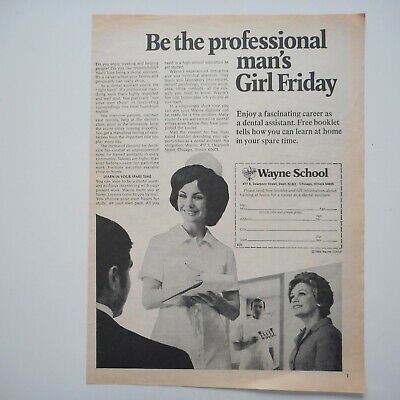This weathered and somewhat faded 1960s magazine or newspaper page, tinged with a brownish hue around its edges, showcases an advertisement for the Wayne School. The page rests on a contrasting black background, highlighting its age and discoloration. Dominating the top right, in large, bold black lettering, is the headline: "Be the Professional Man's Girl Friday." Beneath this, in tiny, nearly illegible black print, clusters several small paragraphs. 

At the center of the page, an image features a woman with straight, short black hair, adorned in a white hat and dress, holding a pad and pencil. She smiles at a man viewed from behind, identifiable by his neatly combed hair and black suit with a visible white shirt collar. To the right of this central image, a sign-up box boldly labeled "Wayne School" promises readers further information. Accompanying this box are photographs of women in professional attire, one possibly a nurse or dental assistant, illustrating the promising careers advertised.

Smaller text details the opportunity to "enjoy a fascinating career as a dental assistant" and invites readers to obtain a free booklet to learn more about training at home in their spare time. In the background, a man in a dental or doctor's outfit observes, adding context to the career paths promoted by the advertisement.